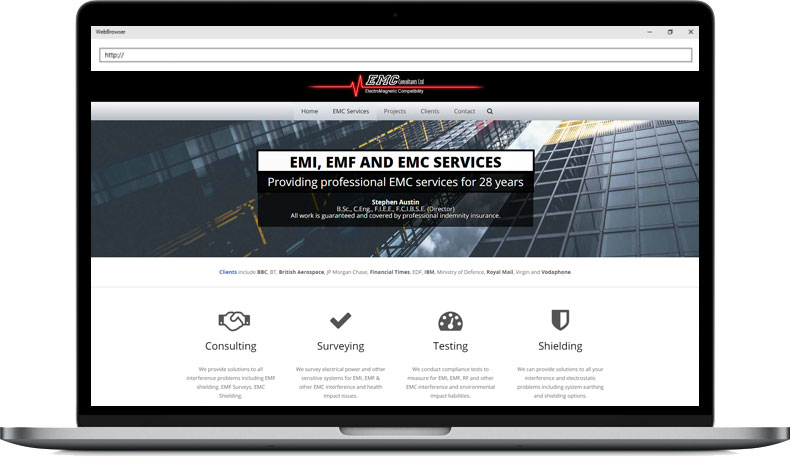This is a detailed caption for an image depicting a screenshot of a website on a computer monitor:

---

The image is a screenshot of a website displayed on a computer monitor, identifiable by the surrounding black bezel and the base of the monitor visible at the bottom. At the very top of the screen, the web browser interface is apparent, featuring an address bar that reads "http://".

The website's main content includes a prominent black and white box centrally placed over a background image. The background image captures an upward view from the base of several skyscrapers, angled dramatically towards the sky. Inside the box, text advertises "EMI, EMF, and EMC Services – Providing Professional EMC Services for 28 Years."

Below this text, a scroll of clients is listed, including notable organizations such as BBC, BT, British Aerospace, JPMorgan Chase, Financial Times, EDF, IBM, Ministry of Defense, Royal Mail, Virgin, and Vodafone.

The lower section of the screenshot features four icons with corresponding labels and descriptions:
1. Consulting – represented by an icon of two hands shaking.
2. Surveying – symbolized by a checkmark.
3. Testing – depicted with an icon resembling a fuel gauge.
4. Shielding – illustrated with a black and white shield.

Each icon links to additional information about the respective services offered. This rich visual and textual content aims to convey the professional scope and reliability of the EMC services provided.